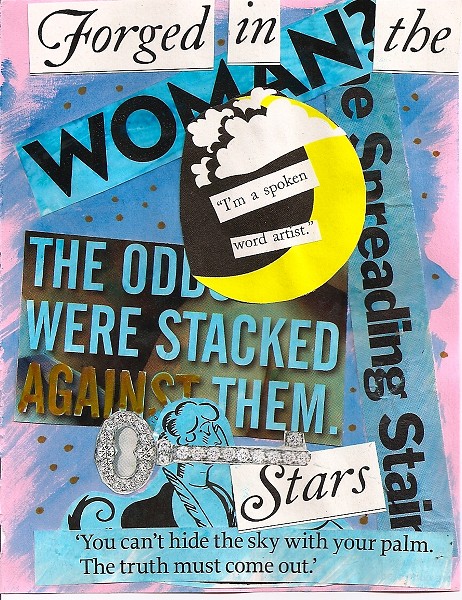The image features a collage art piece set against a pink background adorned with light blue paint smears and brown dots. At the top of the page, there is a white border with bold black text that reads "Forged in thee." Immediately beneath this is a horizontal blue rectangle with black text that says "woman?" To the right, a vertical blue rectangle contains the words "spreading stare" in black text. Further down, another blue rectangular cutout declares "the odds were stacked against them" in blue text. Near this cutout is an illustration of a diamond-encrusted key, positioned adjacent to a cartoon image of a woman, possibly writing with a quill. On a white rectangle with black stars, the bottom portion features blue-colored text stating, "You can't hide the sky with your palm, the truth must come out." Dominating the center of the artwork is a yellow crescent moon set against a black sky with white clouds above it. Overlaid on the moon and clouds are white rectangles with black text that proclaim, "I'm a spoken word artist."